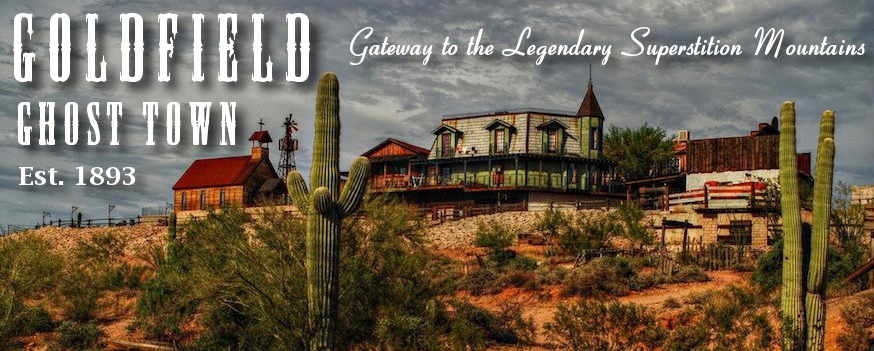A professional, promotional photograph showcases Goldfield Ghost Town, established 1893, as the gateway to the legendary Superstition Mountains. The image is a full-color, horizontally rectangular piece with bold, rustic white text in the upper left, reading "Goldfield Ghost Town, EST. 1893," accompanied by cursive text declaring "Gateway to the Legendary Superstition Mountains." The backdrop is an ominous, cloudy gray sky, setting a dramatic tone. The foreground features reddish sandy soil dotted with green shrubs and towering cacti, some standing between six and ten feet tall with distinctive curved branches. Central to the scene, an old yellowish-brown church with a red roof, white windows, and a cross punctuates the eerie landscape. A windmill rises beside it, adding to the rustic charm. Adjacent to the church, an abandoned inn or large ranch structure—painted in green, brown, and white hues—adds to the wild west allure. The overall theme of the photo captures the essence of a historic ghost town against the rugged, legendary mountains, devoid of any human presence.